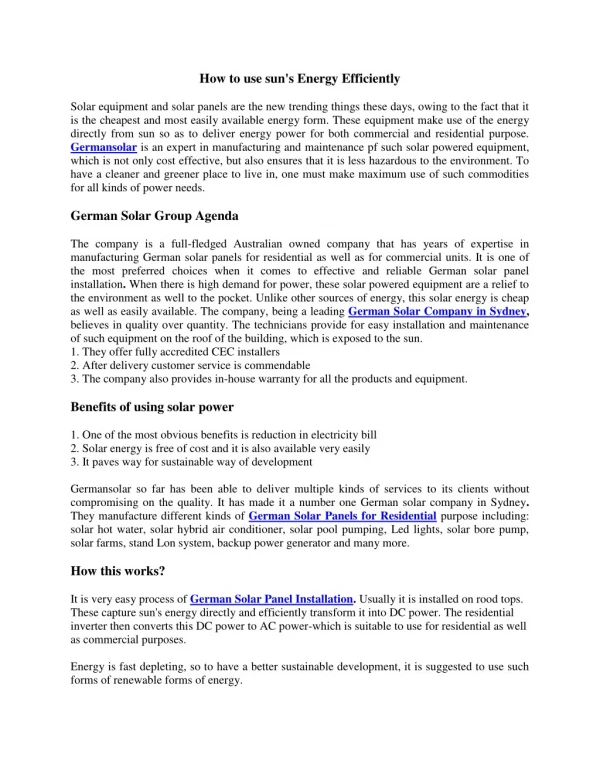The image is a textual document with a rectangular layout, taller than it is wide, displayed on a white background. At the top center of the document, the title "How to Use Sun's Energy Efficiently" is prominently featured in dark lettering.

Beneath the title is a paragraph of black text that spans six and a third lines. On the fourth line of this paragraph, the phrase "German Solar" is distinctively highlighted in purple, underlined, and written in purple ink. This paragraph is block-justified, presenting a sharp, even alignment on both the left and right margins.

Following this paragraph, there is a heading in black text aligned with the left margin that reads "German Solar Group Agenda." Directly below this heading is a new paragraph consisting of seven and a half lines. Notably, on the sixth line of this paragraph, the phrase "German Solar Company in Sydney," is also underlined and written in purple.

Underneath this paragraph are three sequentially numbered lines (1, 2, 3), all flush against the left margin. The text is block-justified, maintaining sharp edges on both sides.

After another space, there is a new section titled "Benefits of Using Solar Power." Following a space after this heading are three numbered lines, each line stacked one on top of the other. Below this, there is another paragraph of text, four and two-thirds lines long. Midway through the third line of this paragraph, the phrase "German Solar Panels for Residential" appears, underlined and in purple, with two additional words following it.

Below this paragraph, a space precedes the next heading: "How This Works?" in black text. Following another space is a paragraph spanning three and a third lines. Directly underneath, there is a continuation of text in another one and a half lines. The first line of this paragraph begins with "It is very easy process of," followed by the phrase "German Solar Panel Installation," which is underlined and written in purple.

Each section and paragraph adheres to a well-organized format, ensuring clarity and easy reading.